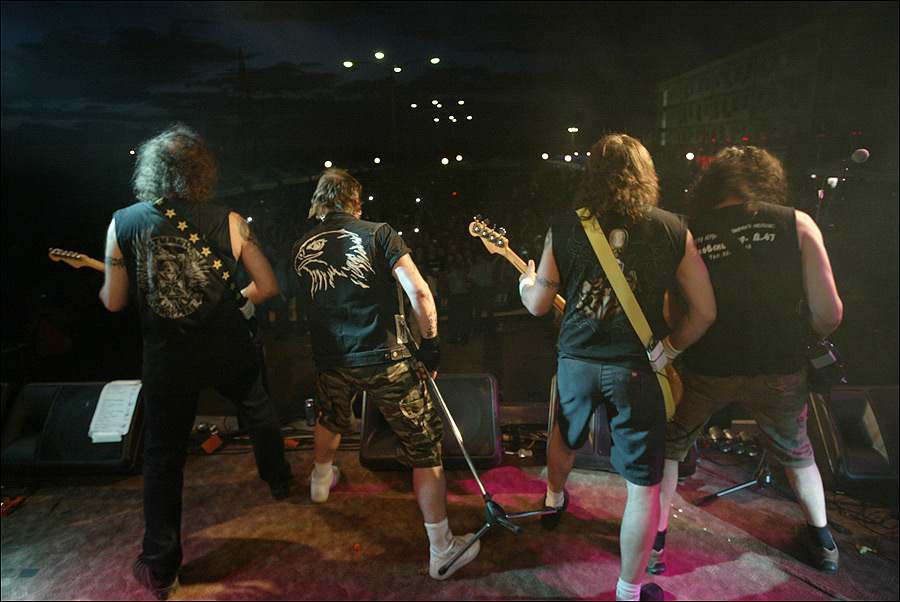In this nighttime outdoor concert scene, a rock band with four members is captured from behind as they perform on a stage with a dark sky filled with ominous clouds above. The stage, lit with purple and pink lights, stands out against the night sky. Multiple streetlights with white lights pierce the darkness in the distance, casting a subtle glow on the large crowd that watches in the shadows in front of the stage. The stage floor appears dark with spots of pink lighting, creating an energetic atmosphere.

The band consists of four male musicians, each in a dynamic, forward-leaning posture. On the left, a guitarist with a shoulder-length shaggy mane and a starred guitar strap wears a short-sleeve shirt adorned with an eagle logo. Next to him, the lead singer grips a microphone stand, dressed in camo cargo shorts, a black t-shirt, and a denim vest featuring an eagle design in white. The third member is another guitarist, distinguishable by his bright yellow guitar strap. He dons black shorts, white socks paired with black shoes, and a sleeveless black t-shirt with an unclear image on the back. The fourth band member, positioned on the right, also wears a sleeveless black t-shirt with unreadable white writing, gray shorts, and has his guitar obscured from view.

Various black amplifiers and speakers line the front of the stage, facing the band. Among the equipment, a piece of white paper is taped to one of the amplifiers, although its writing remains undecipherable. The scene is a vivid snapshot of the band’s pulsating energy and the audience's anticipation, all framed against the dramatic canvas of the night sky.